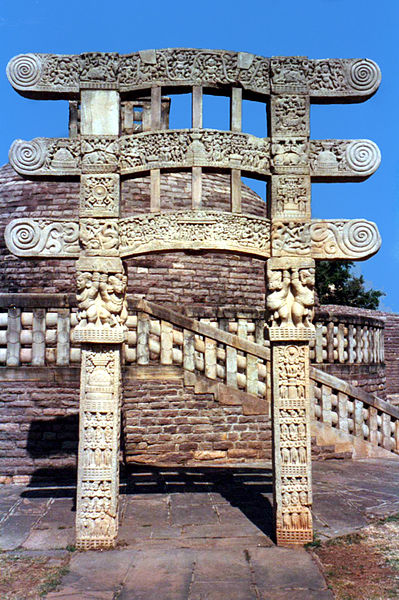The image showcases a majestic, ornate stone structure that stands prominently in front of an ancient temple-like building. The intricate design features numerous swirling patterns and a series of hand-carved figures, including large gargoyle-like characters on the right and representations of an angel and a devil on the left. The structure, which appears to be made up of multiple stone pieces, stands about 15 feet tall and resembles a grand gateway, open to reveal the backdrop. The temple behind has a staircase or ramp leading up, with stone handrails. Beyond the temple, the sky is a brilliant blue, unmarred by clouds, and healthy trees with dark green leaves frame the scene. This photograph exudes an air of ancient civilization, potentially reminiscent of a historic site you'd encounter in regions like South America or Asia, echoing the grandeur of the Seven Wonders of the World.